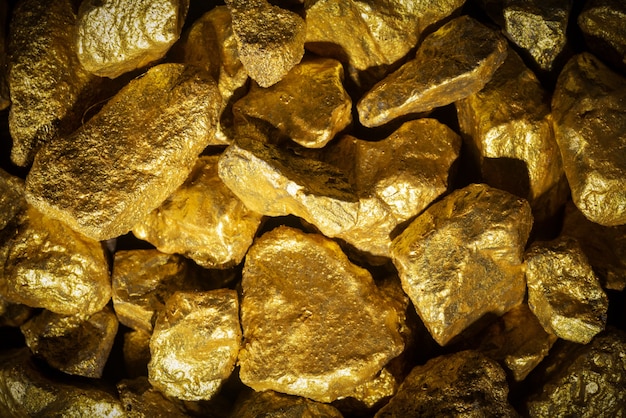The image displays an extensive, close-up view of numerous gold nuggets scattered across the entire frame. These nuggets, varying in shapes and sizes, fill the image completely without any text or additional objects in sight. The nuggets appear to be both small and rounded, as well as slightly larger and more angular, creating a diverse and intricate assembly. They lay in various positions, creating a pile that resembles a mix of rocks, and the bright, well-lit setting enhances their golden color, making the scene vivid and clear.